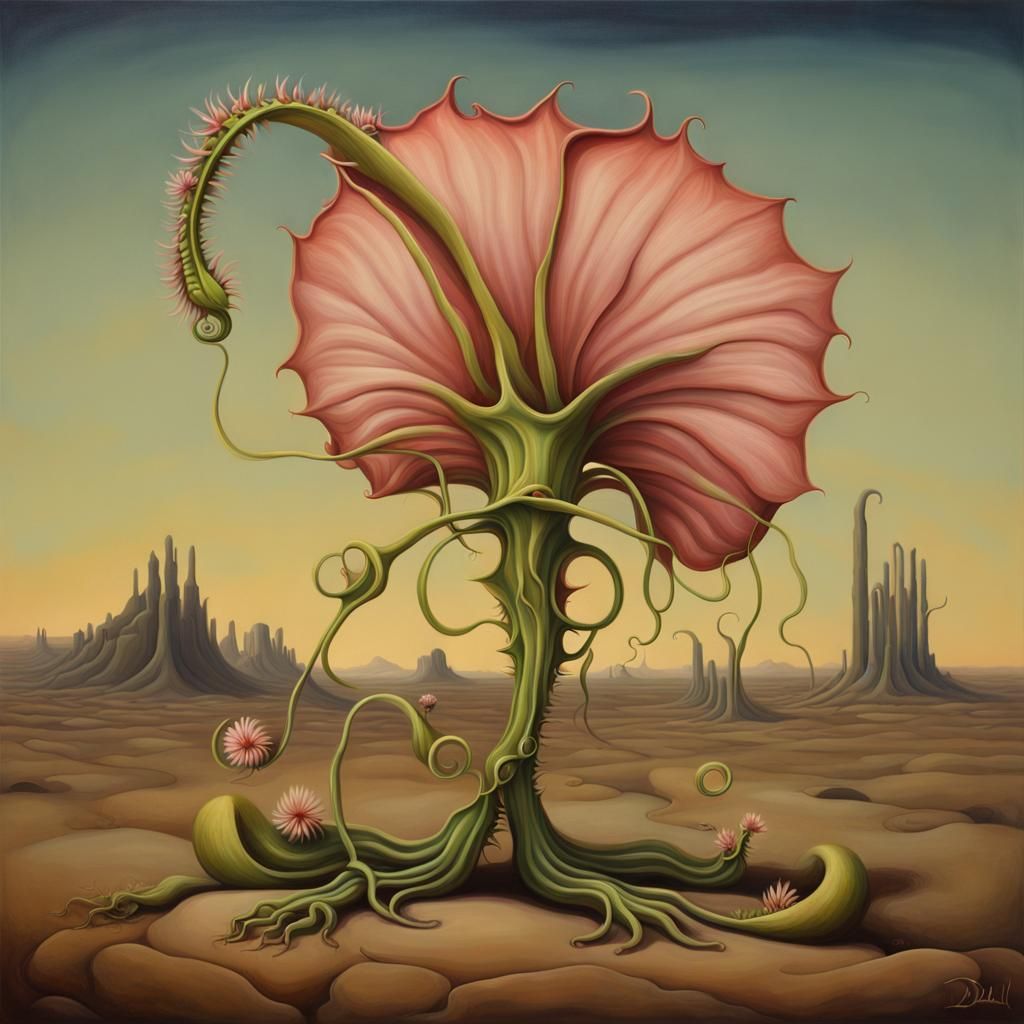The image is a digital illustration of a barren, drought-stricken planet characterized by its dry, cracked ground and devoid of water or life, save for one peculiar and vivid plant-like creature. In the foreground stands this strange plant, its green roots splayed and curling like tentacles upon the dry earth. Rising from these roots is a stem adorned with tiny pink spikes, leading up to a fleshy green leaf. Flanking either side of the stem are tendrils and two leaf-like structures that could resemble feet, giving the plant an alien, almost animalistic appearance. The plant unfurls into two large, pink petals that spread open and stand flared, reminiscent of wings. Adding to its monstrous aspect, nestled within the plant are spiny pink balls, possibly seedlings. This lone plant contrasts sharply with the desolate background of jagged, grey stone outcroppings, evoking an eerie, otherworldly beauty in an otherwise lifeless landscape.